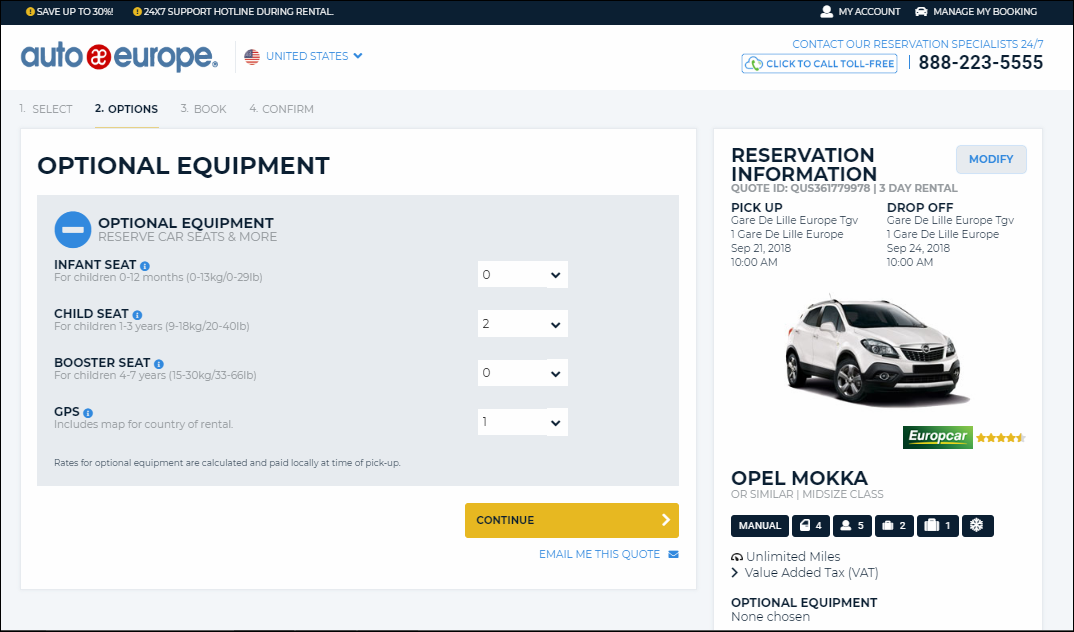The image features a predominantly navy-blue and white-themed graphic with important details for managing a car rental booking through Auto Europe. At the top left, there is a navy-blue circular icon with a white exclamation point, followed by a message in white text that reads, "Save up to 30%." Adjacent to this, another navy-blue circle features the text "24/7," indicating around-the-clock support during the rental period.

On the right side, a white card labeled "My Account" is prominently displayed with the option to "Manage My Booking." The background of this section is a light white color, giving it a clean and professional look. Below, there is a blue banner with the Auto Europe logo, reading "Auto Europe" along with "United States" and an accompanying American flag in a circle.

Further details include a prompt to "Contact our reservation specialist 24/7" in blue, followed by "Click to call toll-free" with the number displayed in black: 888-223-5555. The left side of the image transitions to a gray background featuring a step-by-step guide. Step 1 in gray says "Select," and in black, Step 2 indicates "Optional Equipment."

A white rectangle outlines optional equipment choices such as car seats and GPS units, listed with their respective availability: "Child seat 0," "Booster seat 0," and "GPS 1." It mentions that optional equipment is reserved and paid locally at the time of pick-up.

At the bottom, a mustard-colored rectangle with black text says "Continue," and beside it, a blue link prompts to "Email me this quote." Additionally, reservation information is provided with the quote ID number "QUS361779978" for a 3-day rental.